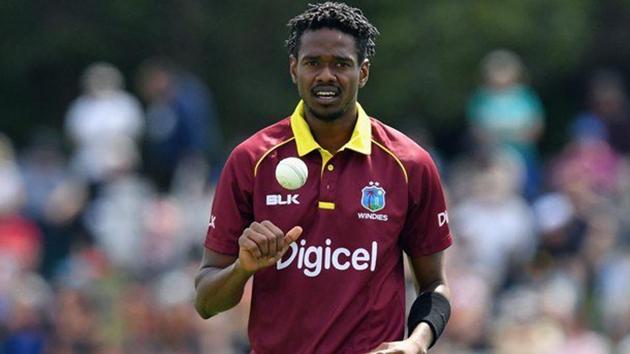This image captures a moment from an outdoor event featuring a male athlete, likely a soccer player, given his attire and setting. He is wearing a distinctive lavender, short-sleeved jersey with a yellow collar. The jersey prominently displays the sponsor name "Digicel" in large white letters across the front. Above the Digicel logo, on the left chest area, there is a "BLK" logo. On the right chest, there's a "WINDES" logo, which is shield-shaped with a blue background and a tropical tree at the center. The athlete, who has dark skin, has dark hair styled in short dreadlocks, and sports a mustache and a small beard. He also wears a wristband on his left forearm. His right hand is raised in the air, suggesting motion or a celebratory gesture. The background of the image is blurred, revealing a crowd of spectators dressed in various colors, likely indicating an enthusiastic audience. Behind them, green foliage and trees are partially visible, adding to the sense of an outdoor setting. There is some ambiguity regarding a ball, but given the context and attire, it leans more towards a soccer player preparing for or after a game.